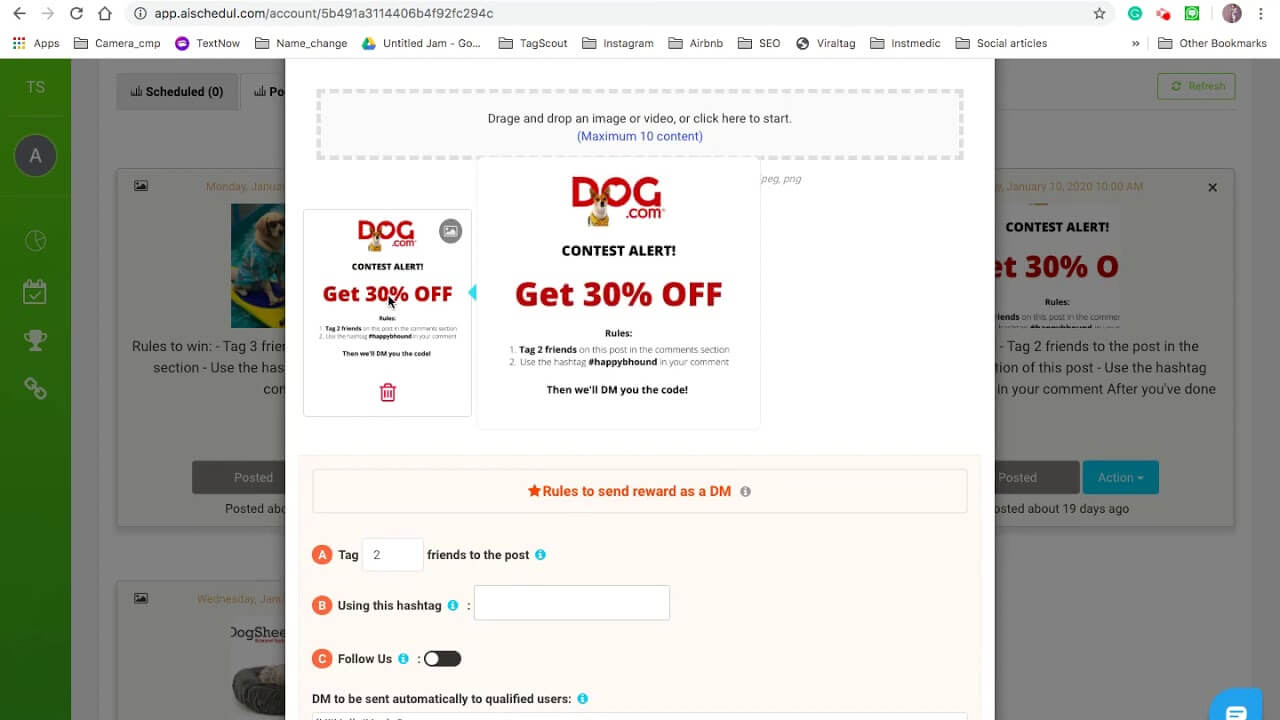This is an intricate screenshot of a browser window displaying the website app.alschedul.com. The full browser interface is visible, including the bookmarks bar. The website is positioned on an account page, displaying a large account number prominently. The user’s account, denoted by the initials "TS" and an icon labeled "A" against a green background, is shown along the left-hand column of the screen.

In the main content area, there are elements related to a contest. Among these are contest rules that include tagging three friends. Adjacent to these details are images featuring dogs and promotional sheets, likely related to the contest. Additionally, a significant pop-up message overlays the screen with instructions: "Drag and drop an image or video or click here to start." This pop-up is part of a larger promotion from dog.com, which advertises a contest offering a 30% discount.

Detailed instructions provided in the pop-up specify the rules for participation:
1. Tag two friends in the post’s comment section.
2. Use the hashtag #HappyBeeHound in your comments.
3. Detailed instructions underneath, highlighted in orange with a star, reiterate the rules for sending rewards via DM, stating:
    - A: Tag two friends.
    - B: Use the specified hashtag (which is not stated explicitly here).
    - C: Follow the account to automatically receive the code via DM.

The screenshot's layered information offers a comprehensive view of user instructions, contest details, and visual elements related to the promotional event.